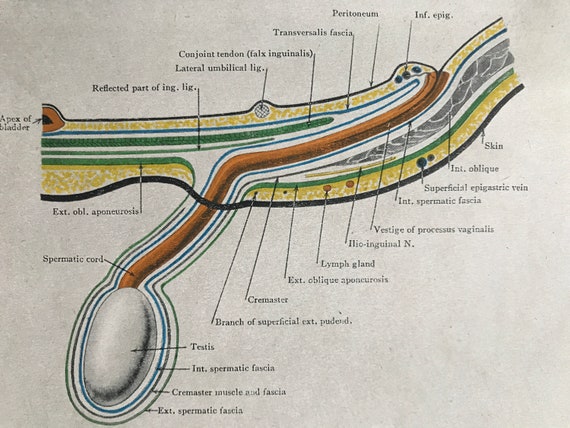This detailed diagram from a physiology book illustrates the internal anatomy of the male reproductive system, focusing on the abdomen and testicular region. Set against a gray background, the diagram labels various anatomical structures with thin black lines pointing to corresponding parts. Prominent elements include the conjoint tendon, lateral umbilical ligament, and transversalis fascia, indicating layers of the abdominal wall. The image also highlights the lymph gland and interseptic forcula, with blue and green lines marking the veins and surrounding tissue.

The diagram provides a sideways view of the male genitalia, with the testicles positioned at the bottom left and the penis extending towards the upper right. The testicles are depicted as white, egg-shaped structures enclosed by layers such as the external fascia and cremaster muscle. The spermatic cord is also labeled, along with the epigastric vein and peritoneum, the latter depicted in a yellow layer around the abdominal wall. This complex illustration serves as an educational tool for understanding the intricate connections and layers within the male reproductive and abdominal regions, particularly in the context of explaining hernias.